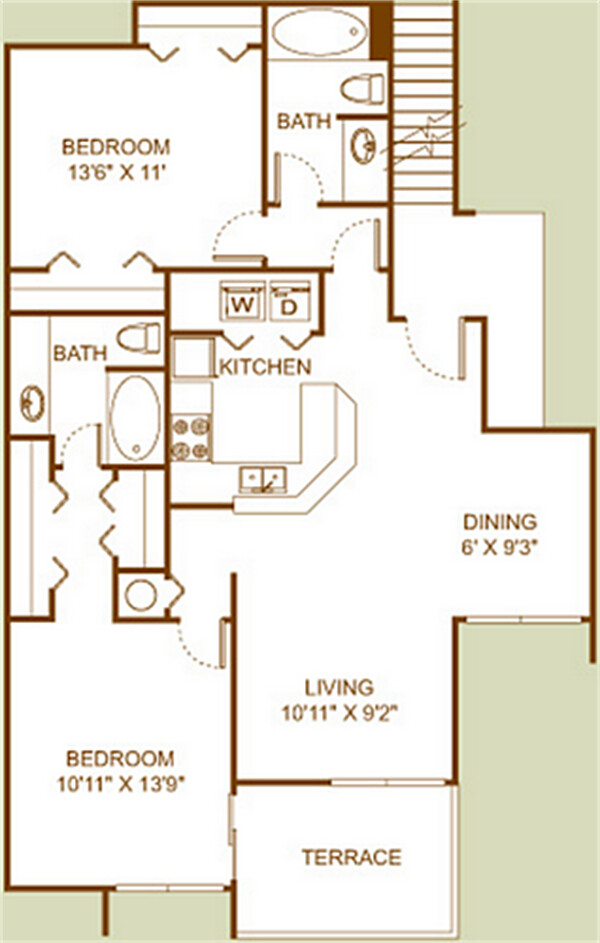This detailed floor plan depicts a first-floor unit within an apartment building or condominium. The layout is predominantly rectangular but features several cutouts, especially along the right-hand side, creating an irregular shape. A notable square jut-out is present, adding further complexity to the design.

Upon entering from the front, there is a bedroom immediately visible, accompanied by a terrace that offers outdoor space. The central living area comprises an open floor plan that seamlessly integrates the kitchen, dining, and living room, fostering a spacious and unified living environment. The dining area prominently juts out, adding character to the space. 

The kitchen is equipped with modern amenities, including a washer and dryer. Towards the back, a second bedroom and a separate bathroom can be found. A wall and a set of stairs distinctly divide these areas, ensuring privacy.

The front bedroom, designated as the master or primary bedroom, features an en-suite bathroom and a closet, enhancing convenience and luxury for its occupants.